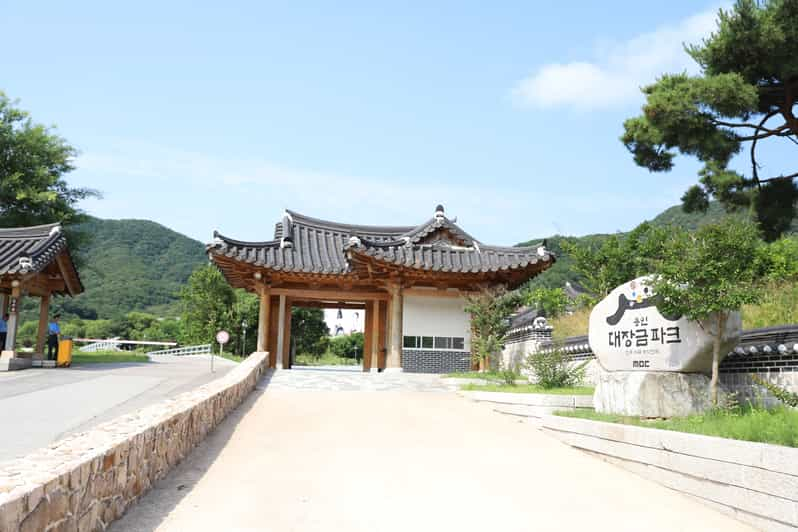The photograph captures an outdoor scene featuring an entry gate to a town or temple, likely located somewhere in Asia. The image is taken from the perspective of someone approaching the gate on a wide stone, tan-colored path that ascends slightly uphill towards the pagoda-like structure. The pagoda boasts two entrance portals supported by wooden posts and a traditional black tile-style roof with upward-sweeping edges, embodying an authentic Asian architectural design.

To the right of the path, a cement-style wall runs alongside, while on the left, a low stone wall parallels the path leading up to the entryway. Prominent in the scene is a large rock adorned with Chinese characters, positioned under a big green tree. The background showcases gently rolling hills blanketed in greenery and dotted with additional trees, adding to the tranquil, picturesque setting. The sky above is a soft, light blue with delicate, wispy clouds, suggesting a sunny day. This comprehensive view indicates the entrance might serve either as a tollway or as an access point to a park or cultural site.